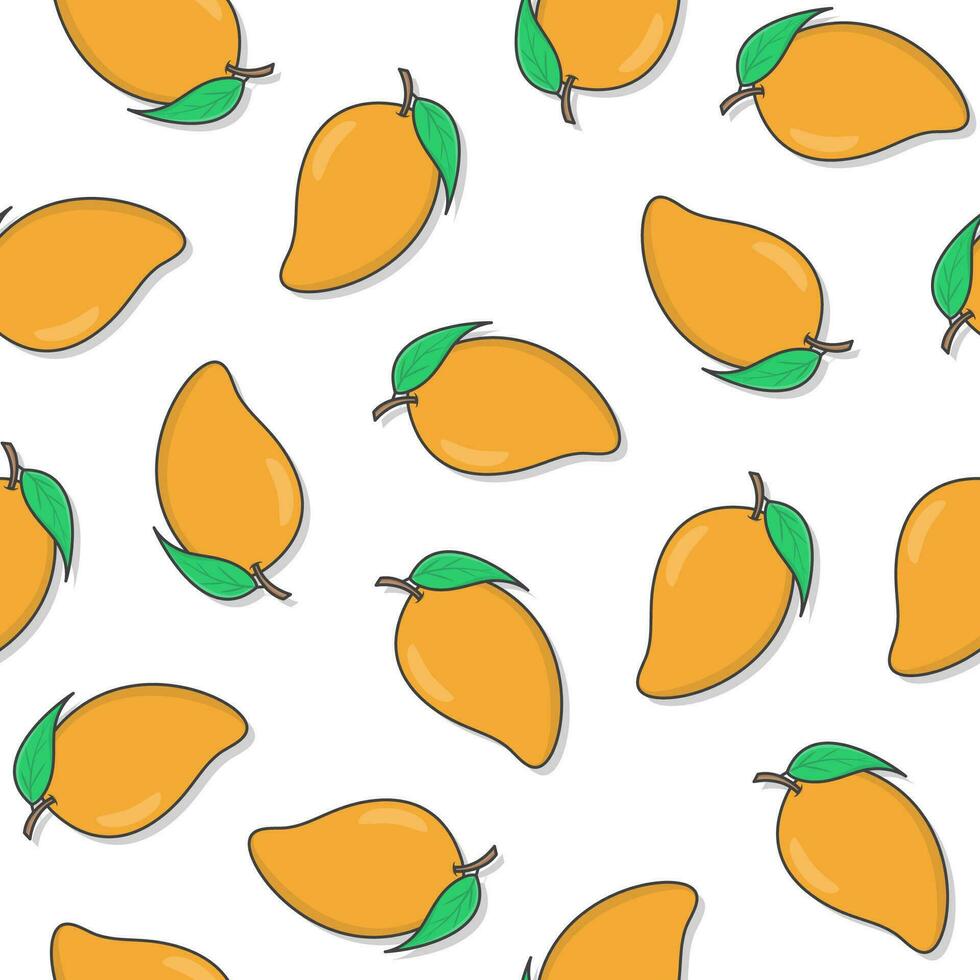This is a detailed, cartoon-style animated drawing of 19 orange-hued fruits, possibly mangoes, set against a white background. Each fruit features a brown stem and a single green leaf, with the highlight on the leaf showing some veining details. The predominantly golden-orange fruits, all identical, are depicted in various rotations—some facing upwards, sideways, or downwards. The fruits are arranged in a slightly topsy-turvy manner, with a few extending beyond the frame, making them only partially visible. Each fruit is highlighted by curved light reflections and subtle shadows beneath them, enhancing their three-dimensional appearance despite the overall stylized and non-realistic representation. All elements are outlined in black, creating a crisp and vivid visual effect.